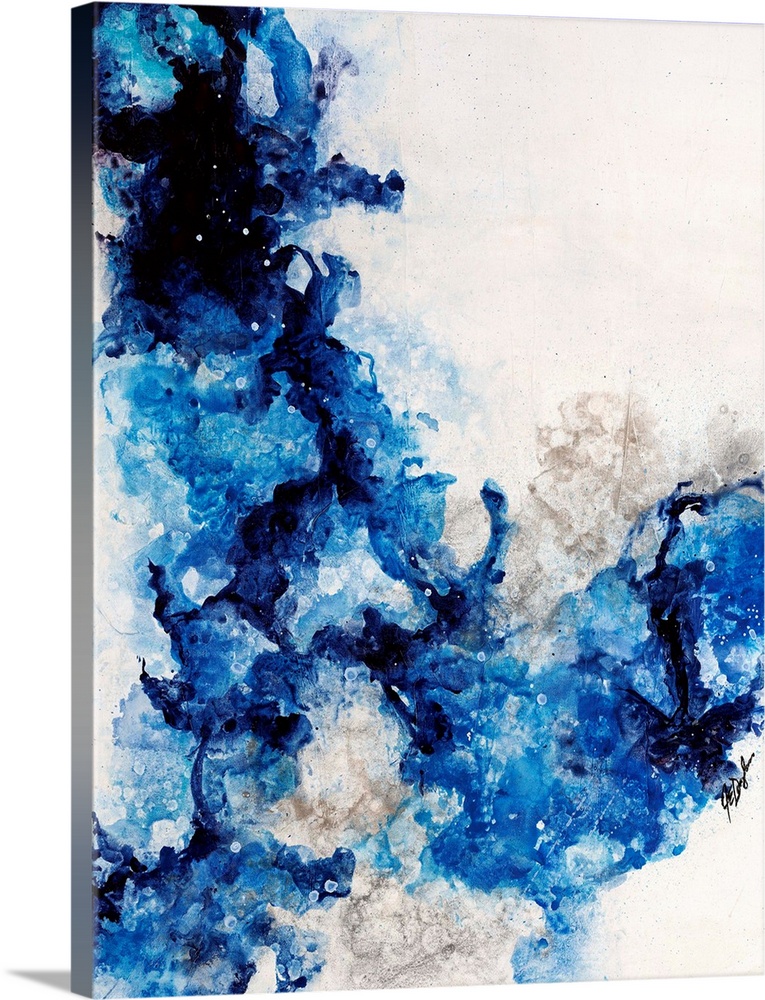This is an image of a vertical rectangular canvas painting, primarily off-white in color. The artwork features a dynamic and abstract design with a splattering of blue, black, gray, and a few tan hues. The paint is predominantly concentrated on the left-hand side and the bottom right quadrant of the canvas, with the upper left corner displaying darker splotches. The design's blue shades range from light to deep, giving a nebula-like appearance, reminiscent of a star cluster. The right upper part and the lower right corner of the canvas remain mostly unpainted, featuring sparse splatters and maintaining the canvas's original white shade. Shadows cast by the canvas itself are evident, emphasizing its three-dimensional quality. Additionally, a hard-to-distinguish signature is present in the lower right-hand corner, subtly nestled among the few white spots that stand out against the painted areas.